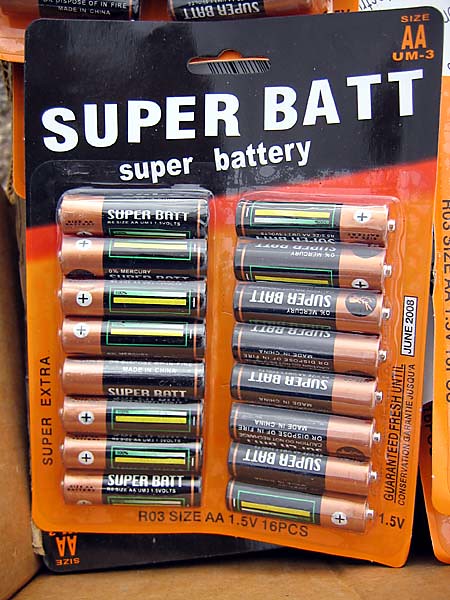The image displays a close-up of a pack containing 16 AA batteries labeled as "Super Bat Super Battery". The packaging features a gradient design, transitioning from black at the top to orange at the bottom, reminiscent of the Duracell brand but potentially a knockoff. In the top right corner, the package specifies the battery sizes as "AA UM-3". Dominating the middle section, the text "SUPER BAT" is prominently written in large white letters, with "Super Battery" beneath it in smaller font. Each individual battery has a gold tip, transitioning to a black body, and is inscribed with "Super Battery" alongside two small power bars colored yellow and light blue. The batteries are arranged in two vertical rows of eight, encased in a clear plastic covering. At the bottom of the package, in black lettering, it states "RO3 Size AA 1.5V 16 pieces". On the right side, it mentions "Guaranteed fresh until June 2008", accompanied by additional conservation details, possibly in another language. Small portions of other packages are visible in the background, featuring similar black and orange color schemes.